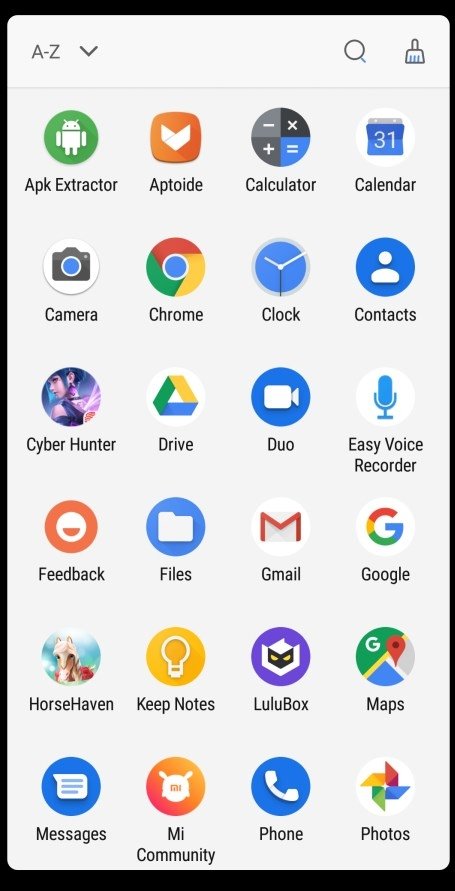Displayed is the app drawer of an Android phone with a light gray background and a simple, clean design. The icons are arranged in alphabetical order, each contained within a circular boundary. Some of the prominent apps visible include APK Extractor, Aptoide, Calculator, Calendar, Camera, Chrome, Clock, Contacts, Cyber Hunter, Drive, Duo, Easy Voice Recorder, Feedback Files, Gmail, Google, Horse Haven, Keep Notes, LuluBox, Maps, Messages, Me, MI Community, Phone, and Photos. 

The drawer features sorting options situated at the top left, allowing the user to organize apps in various ways. Currently, the apps are sorted alphabetically. Additional functionalities include a search icon (magnifying glass) for quickly locating specific apps, and a brush icon, which might be used for cleaning up or hiding apps. Noteworthy is the inclusion of some advanced applications such as APK Extractor, suggesting the phone's user may have rooted their device, granting them lower-level permissions and the ability to install applications from outside the official Play Store.